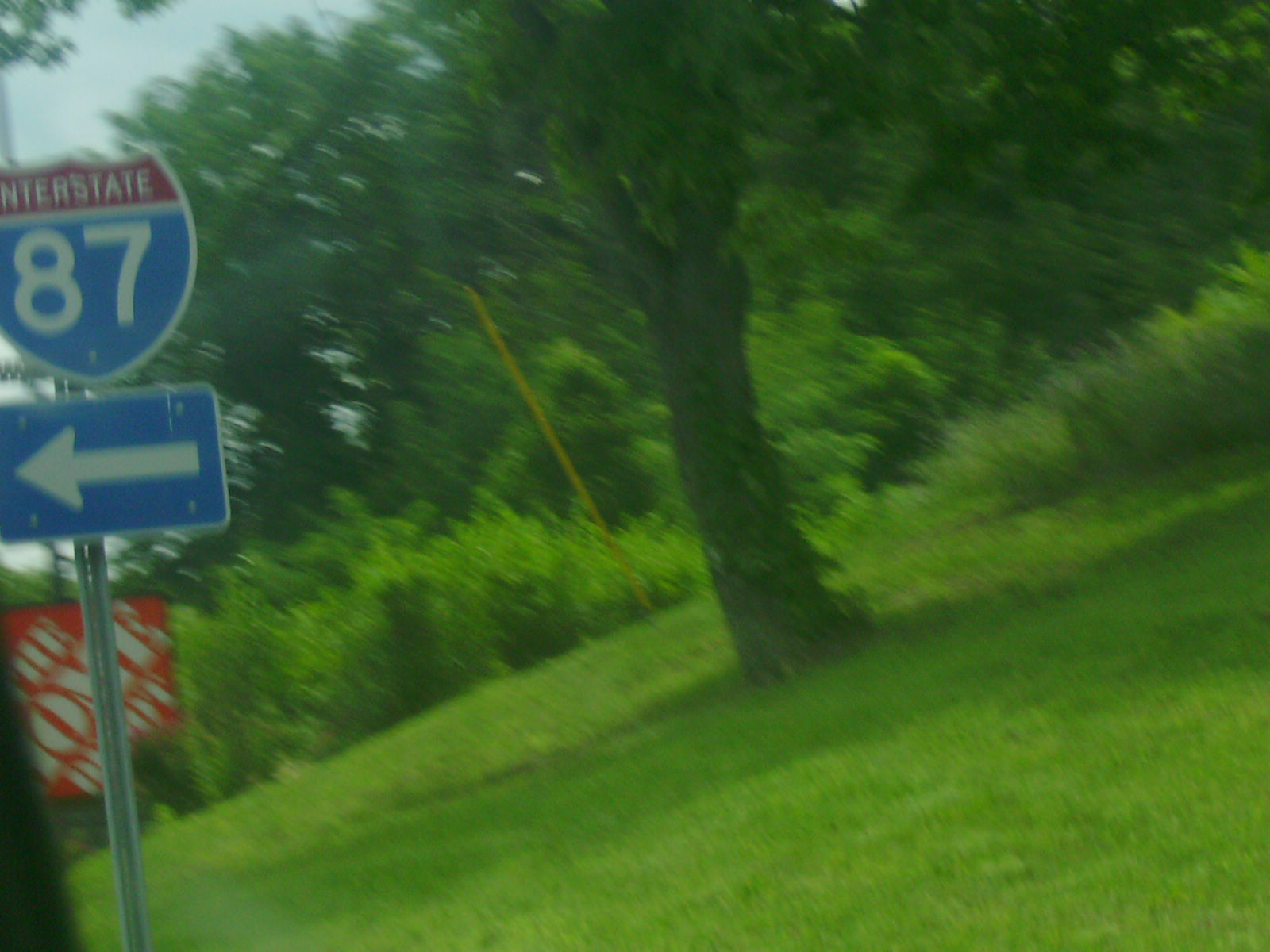This photograph captures a slightly tilted interstate sign for Interstate 87, prominently featuring a left-pointing arrow. The sign itself appears mounted on a silver pole. Behind this pole, there is a partially obscured store sign for The Home Depot, with the pole cutting through its center, making the full sign difficult to see. To the left of the interstate sign, near the lower left-hand corner, there's a noticeable black object. The surrounding environment is lushly green, showcasing a tree with dense foliage and wild green weeds. Additionally, a solitary yellow pole stands behind the primary tree, unattached to any visible structure, enhancing the layered depth of the scene. The tree and other elements seem crooked due to the slanted angle from which the image was taken.